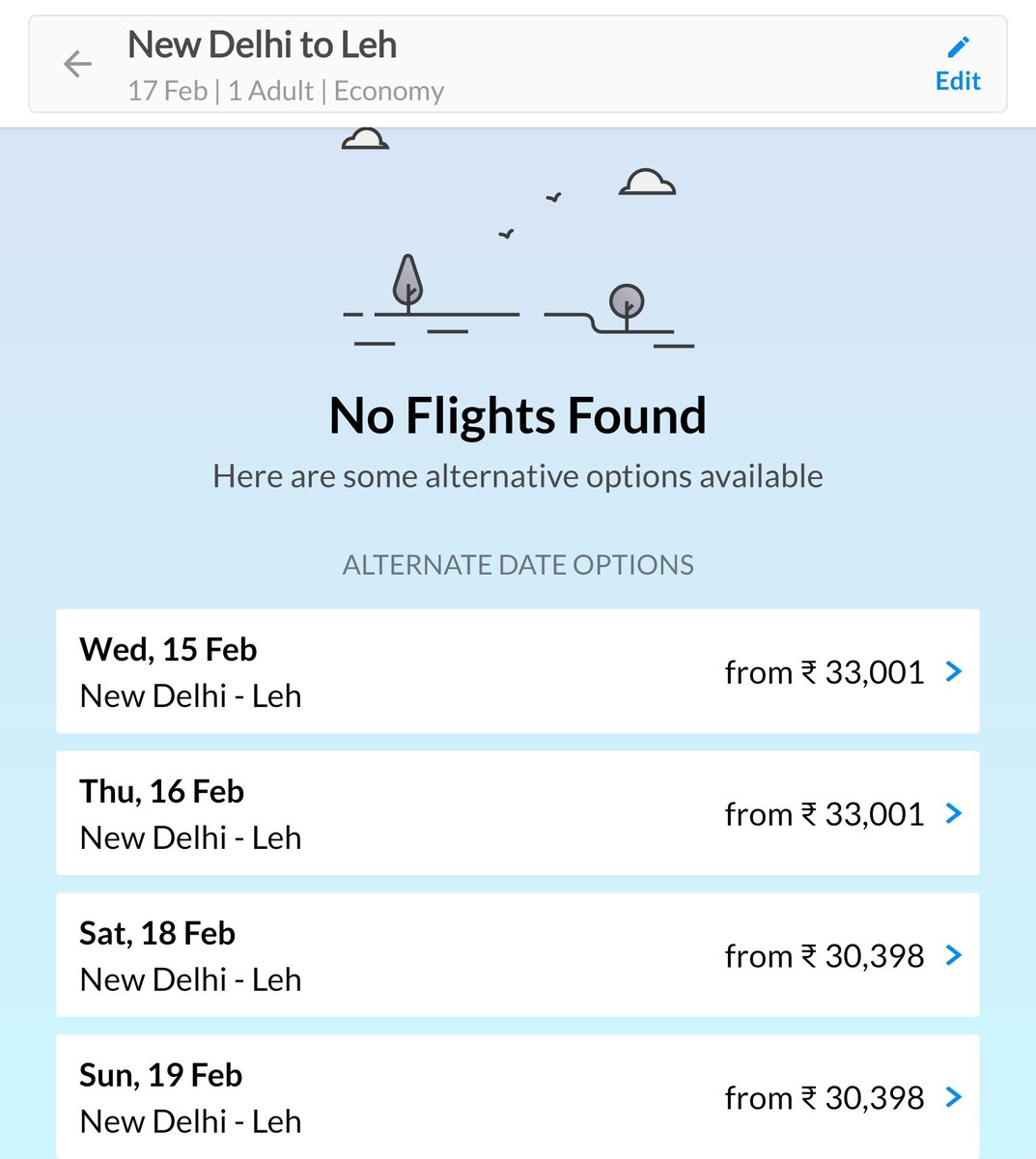The image in question displays a flight search screen with detailed information about flight options. At the top, a gray pane features an arrow pointing left, and in dark letters, it says "New Delhi to Leh, 17th Feb, one adult, economy." Positioned on the right side of this bar, a blue pencil icon accompanies the word "edit." The primary background of the screen is light blue and includes simplistic graphics of a tree, two clouds, and two birds in the sky, giving a rudimentary visual touch.

Directly below the graphics, in bold dark letters, the message "No flights found" is prominently displayed. Beneath this, smaller gray letters provide further context: "Here are some alternative options available." This is followed by another line in gray capital letters: "ALTERNATE DATE OPTIONS." The screen then lists four alternative flight options on individual white panes:

1. Wednesday, 15th Feb, New Delhi to Leh, with prices starting from 33,001 (currency not specified).
2. Thursday, 16th Feb, New Delhi to Leh, also from 33,001 (currency not specified).
3. Saturday, 18th Feb, New Delhi to Leh, starting at 30,398.
4. Sunday, 19th Feb, New Delhi to Leh, beginning at 30,398.